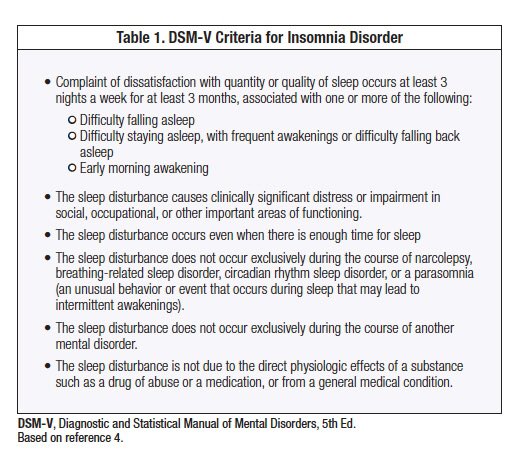In this image, we see a black-outlined box set against a gray background. The first line within the box displays bold black text reading, "Table 1: DSM-5 Criteria for Insomnia Disorder." Following this heading, there is a list of bullet points detailing the diagnostic criteria for insomnia disorder. They state that a complaint of dissatisfaction with the quantity or quality of sleep must occur at least three nights per week for at least three months, and must be associated with one or more of the following conditions: difficulty falling asleep; difficulty staying asleep, characterized by frequent awakenings or trouble falling back asleep; or early morning awakenings. Additionally, this sleep disturbance must cause clinically significant distress or impairment in social, occupational, or other important areas of functioning, and it must occur despite there being sufficient opportunity for sleep. Beneath the outlined box, the text reads, "DSM-5: Diagnostic and Statistical Manual of Mental Disorders, 5th Edition."